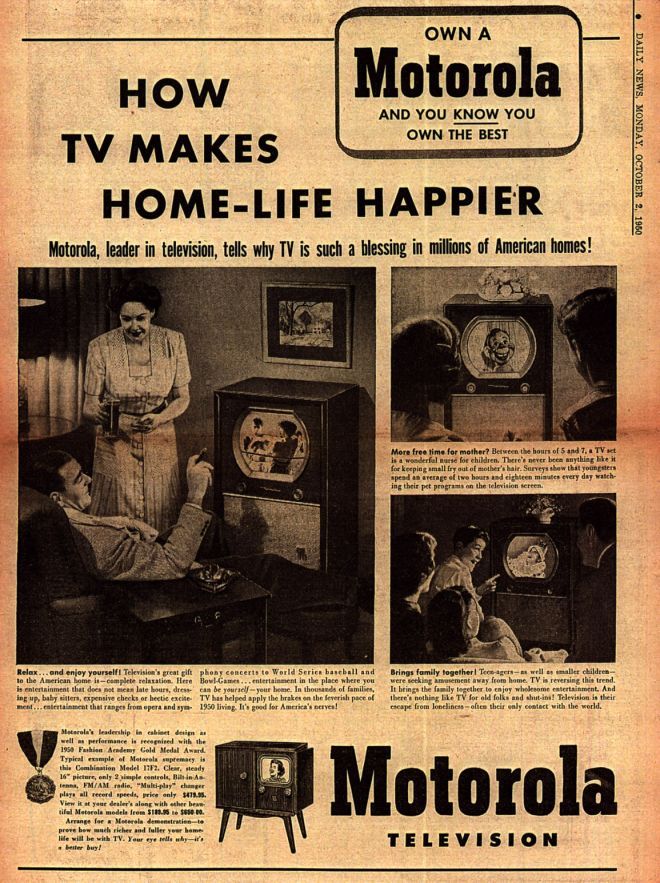This image is an antique advertisement for a Motorola TV, appearing in the Daily News on Monday, October 2, 1950. The headline boldly declares, "How TV Makes Home Life Happier," with the tagline, "Own a Motorola, and you know you own the best." The ad emphasizes Motorola as the leader in television and highlights the joy and relaxation TV brings to millions of American homes. 

The central section of the ad features three photographs. The leftmost picture depicts a man reclining in a chair, smoking a cigar, with a woman standing over him, seemingly about to offer him a drink. Both are focused on the TV. The top right photo shows two children engrossed in a show featuring a puppet, reminiscent of Howdy Doody. The bottom right image captures a group of teenagers watching TV, one of them pointing at the screen which displays a woman.

The ad reiterates the message of television as a source of complete relaxation and joy for the whole family. Below the images, large text reads "Motorola Television" alongside an illustration of a TV console with a lady on the display screen.